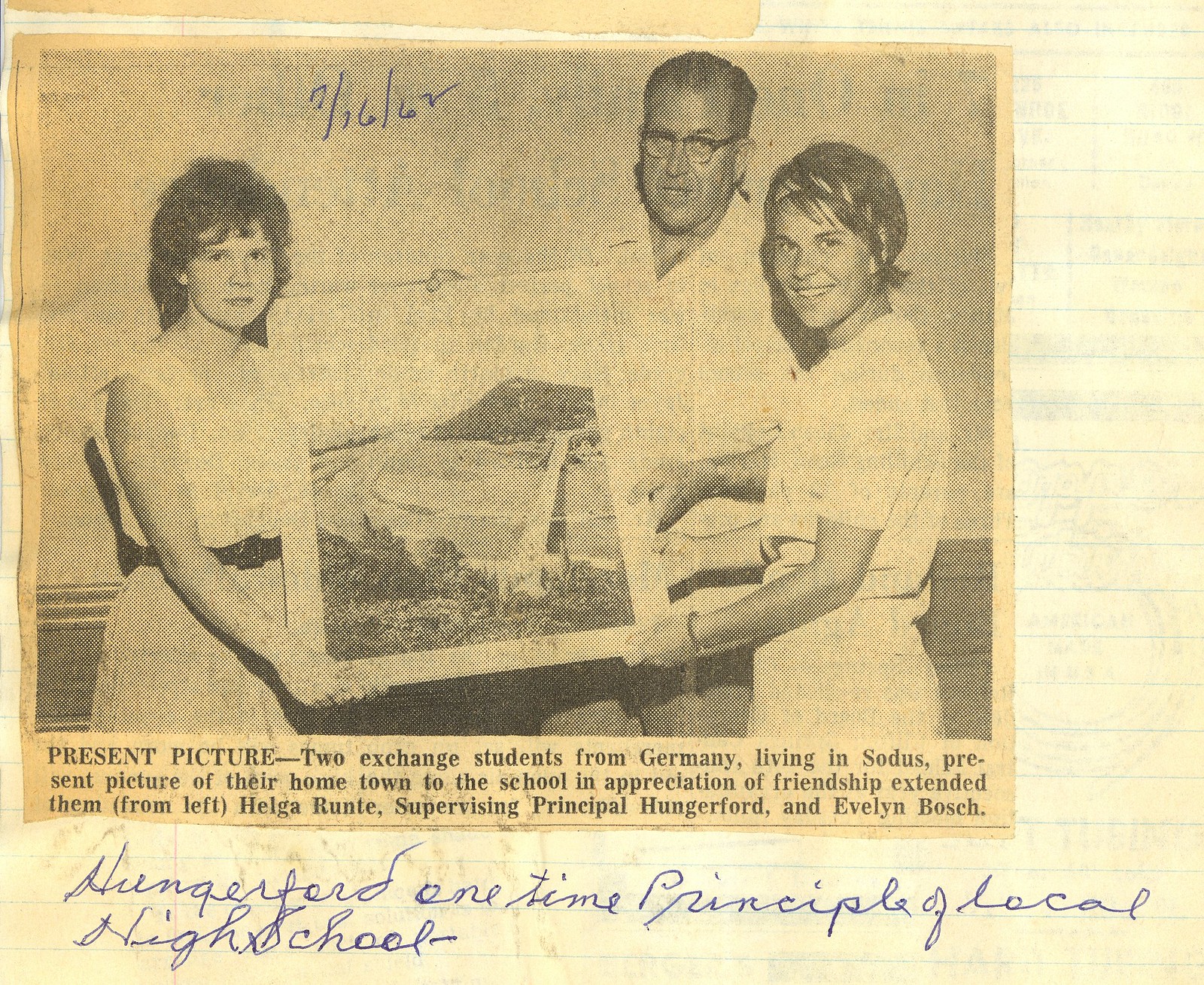This photograph, cut out from a newspaper and mounted on lined paper, dates back to July 16, 1962, as noted in blue ink at the top. The black-and-white image captures two women and a man standing close together and holding a photograph depicting an outdoor scene of a bridge connecting an island to the mainland. On the left, one woman, with curly hair and a black belt, maintains a neutral expression. On the right, another woman with shorter hair smiles, while behind her, a bespectacled man—Supervising Principal Hungerford—stands, also not smiling. A caption beneath the image reads: "Two exchange students from Germany living in Sodus present a picture of their hometown to the school in appreciation of the friendship extended to them." The individuals are identified as Helga Rundt on the left and Evelyn Bosch on the right. Additionally, there is cursive handwriting noting Hungerford as a one-time principal of a local high school.